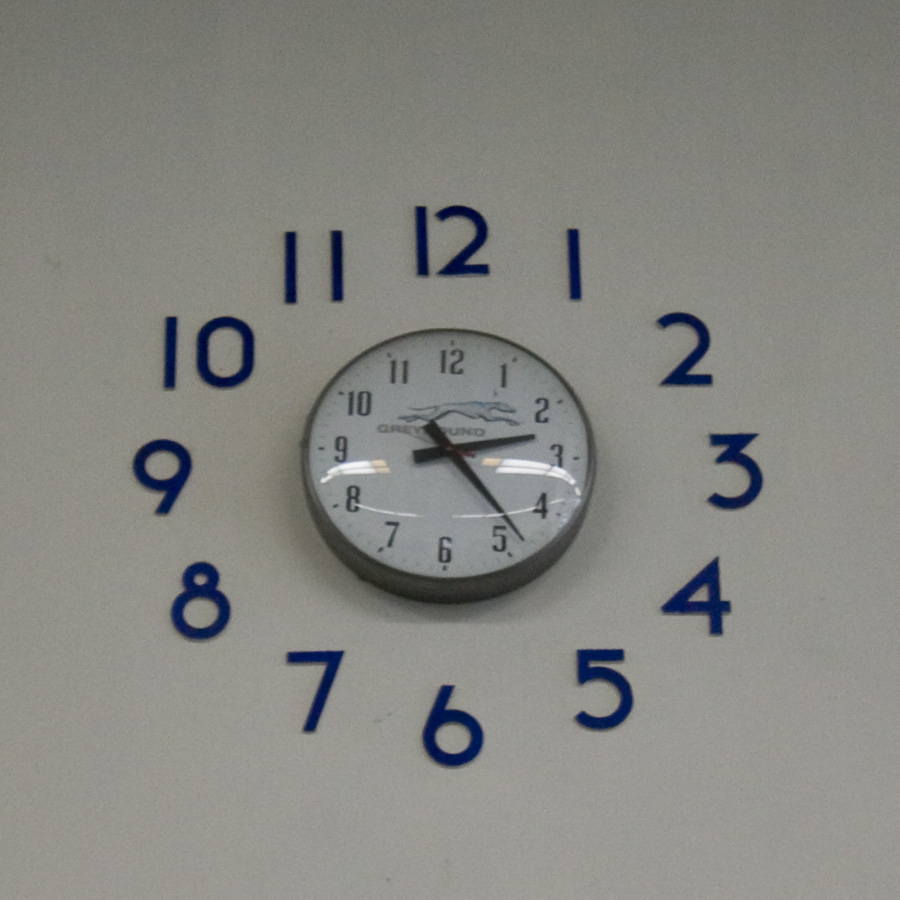The image is an indoor photograph of a clock on a white wall, typical of what might be seen in a classroom. The clock itself has a traditional design with black numbers from 1 to 12 against a white face, framed with either a black or silver border. The minute hand points just before the 5, indicating the time is approximately 2:24, with the hour hand slightly past the 2. Notably, the clock features a graphic of a greyhound dog running across its top. Adding a unique element to the scene, around the clock are large blue numbers adhered directly to the wall. These numbers form a clock-like pattern, with 12 at the top, and descending sequentially, wrapping back up to 12, exactly matching the positions of the numbers on the clock face.